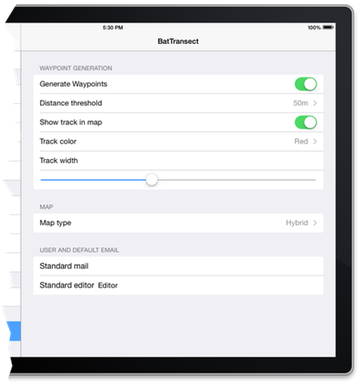The image is a screenshot from a computer display, although part of it appears cropped off on the left side. Enclosed by a black rectangular border that is visible along the top, right, and bottom edges, the left side of the screen shows signs of irregular cropping. At the top of the screen, there is a label that reads "Bat Transect." The battery icon indicates full charge at 100%, and the current time is displayed as 5:30 PM.

Further down the screen, the section titled "Waypoint Generation" includes various configurable options. The feature to "Generate Waypoints" is activated. The "Distance Threshold" is set to 50 meters, and the option "Show Track on Map" is enabled. The selected "Track Color" is red. The "Track Width" is controlled by a slider; currently, the slider indicator is partially blue and set at approximately one-third of the maximum range, with the remaining portion in gray.

Lastly, the "Map Type" is configured to "Hybrid," although additional information beyond this point is not fully visible due to cropping.